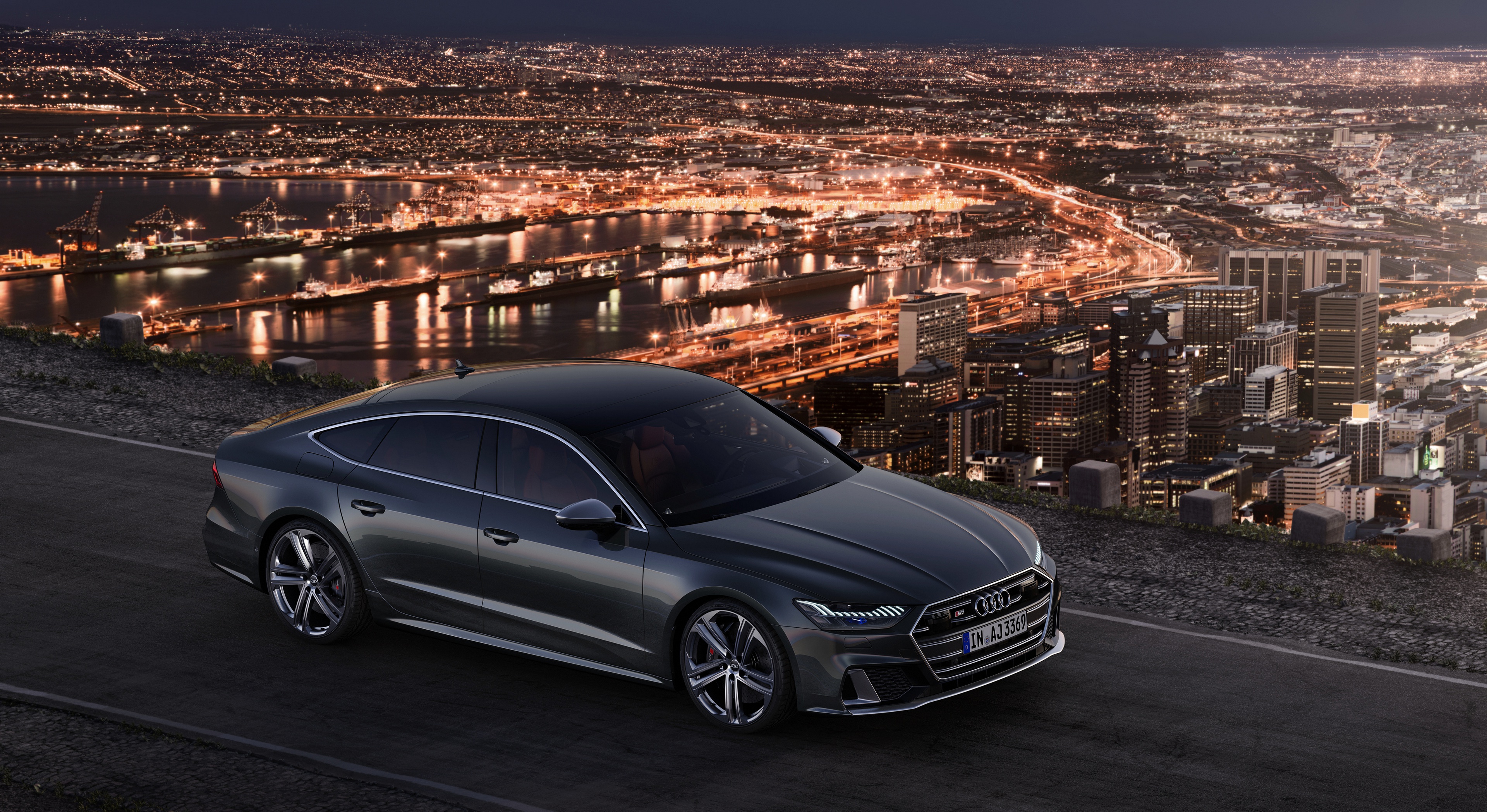A sleek, black Infiniti car with tinted windows is driving on an illuminated road at night, with the striking urban backdrop of a bustling city behind it. The car, which sports a modern and streamlined design, is captured from an angle that emphasizes its front right side as it faces towards the right. The car features two doors and a hatchback-inspired design, although it isn't a true hatchback. The cityscape showcases numerous high-rise buildings adorned with bright, orange-hued lights, which appear to reflect off a large body of water, adding to the vibrancy of the scene. The photo, taken outdoors, beautifully contrasts the dark silhouette of the car against the lively, light-speckled city, evoking a sense of dynamic urban life.